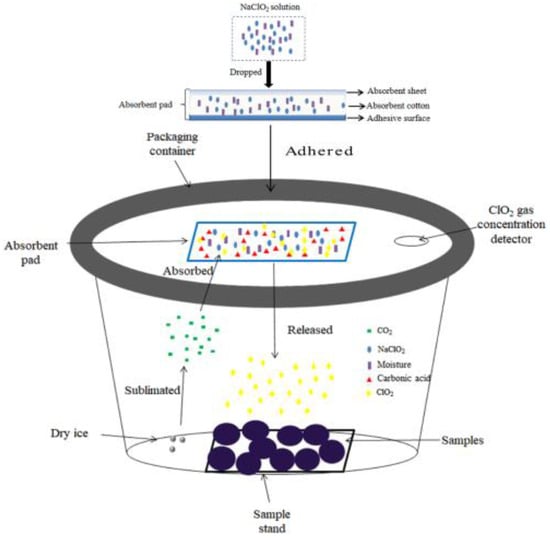This detailed diagram illustrates a cylindrical transparent plastic container with a gray rim, showcasing a complex scientific process. At the top, a NaClO2 solution is dropped through an absorbent pad, which consists of a sheet, absorbent cotton, and an adhesive surface. The pad is attached to the packing container, and various colored dots in the diagram indicate different elements: carbon dioxide (CO2) levels, moisture levels, carbic acid levels. 

Within the container, small blue dots labeled as dry ice reside at the bottom, directly beneath larger purple balls marked as the sample stand. Arrows and a detailed legend on the right clearly explain the elements and their interactions. The dry ice sublimates, releasing gas that moves upward to a concentration detector for ClO2 gas, located above the sample stand. The diagram meticulously represents the flow and interaction of substances within the container, complete with color-coded indicators for easy interpretation.